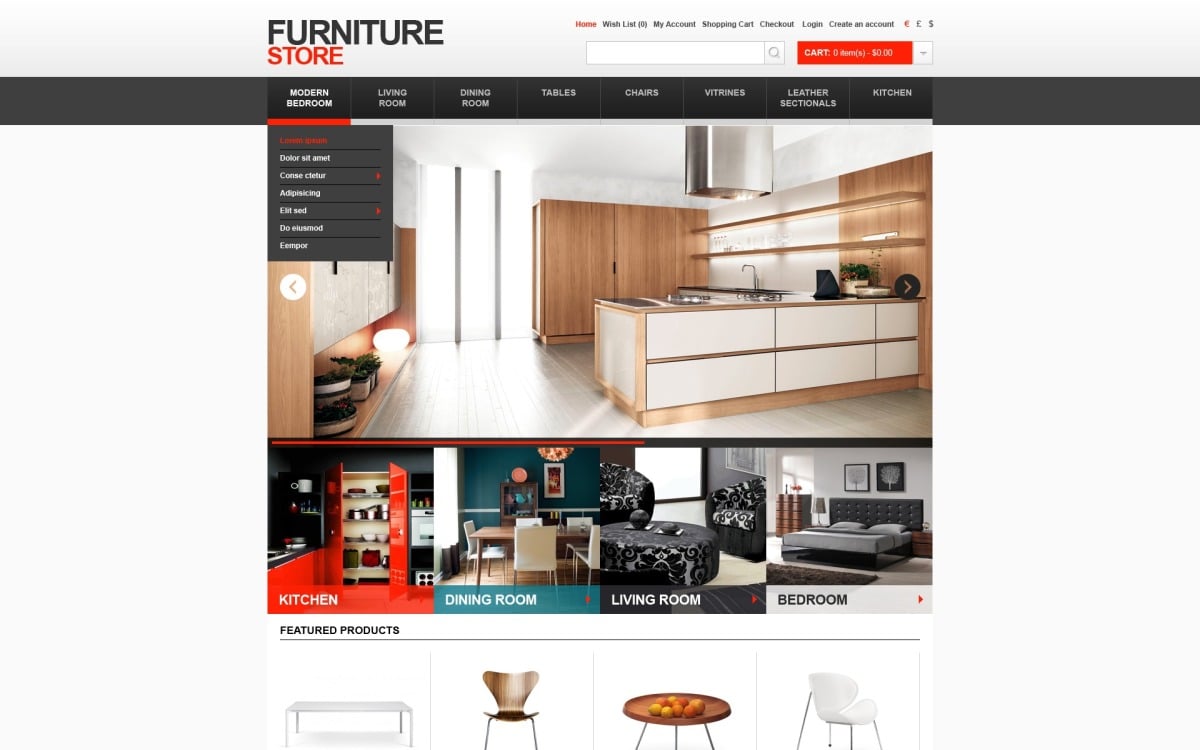The image features a website design with a light gray background. At the top, a header in the same light gray color prominently displays the text "Furniture Store," with "Furniture" in black and "Store" in red. Incorporated within the header is a search bar complete with a magnifying glass icon, positioned against a dark gray backdrop.

Below the header, there's a large image representing a home kitchen. An orange label marked "Kitchen" is situated just beneath the kitchen image. Adjacent to this, a blue label reads "Dining Room," a dark gray label reads "Living Room," and a light gray label reads "Bedroom."

Further down, the section titled "Featured Products" showcases images of various furniture items. This includes a wooden end table, a brown wooden chair, another end table, and a white chair, all neatly arranged to visually complement the descriptive labels above.